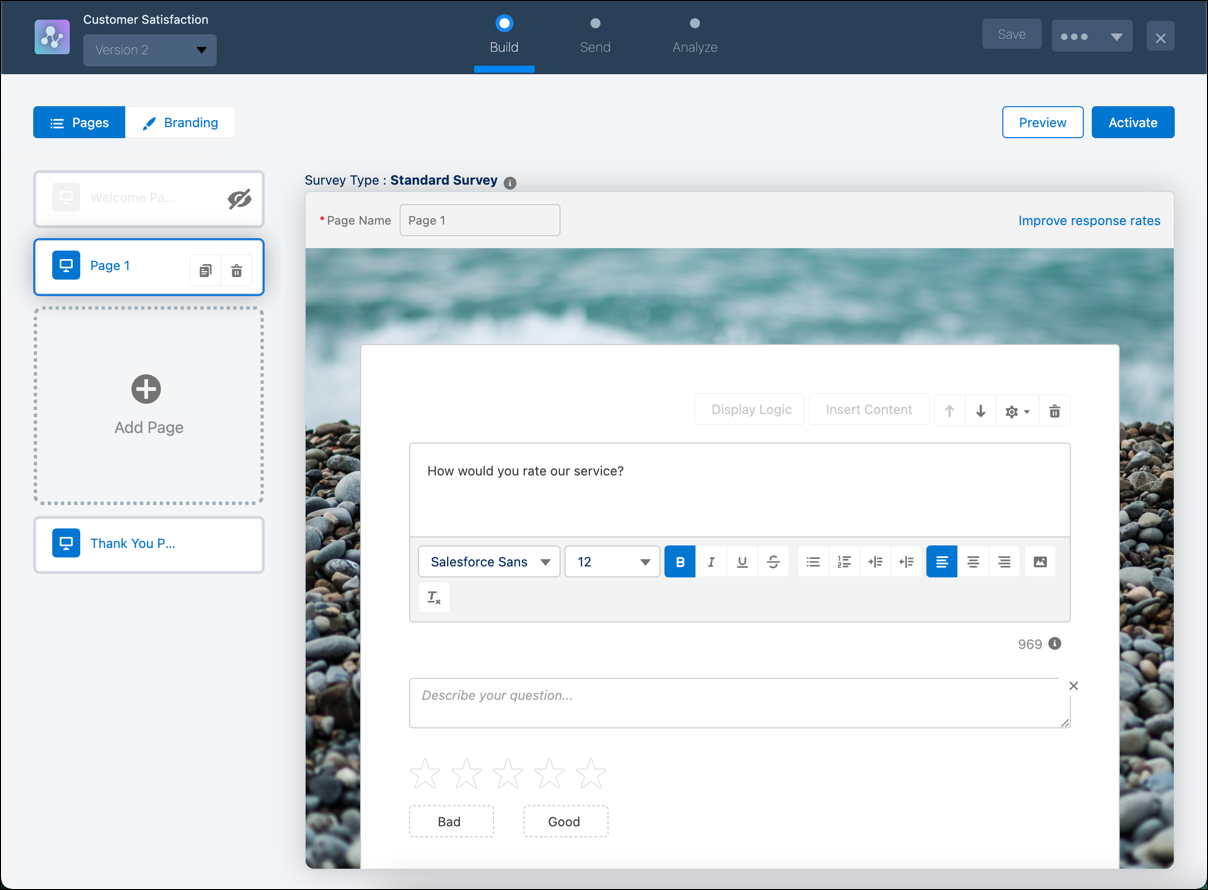The header section of this page features a dark blue background with "Customer Satisfaction Version 2" written on the top left. To the right, three sections, namely "Build", "Send", and "Analyze" are displayed, with "Build" being highlighted and underlined in blue. On the far right of the header, there are options for "Save", a drop-down menu, and a close button.

On the left sidebar, two categories are visible: "Pages" and "Branding". The "Pages" section is highlighted in blue, while "Branding" is written in blue but has a white background. Under the "Pages" section, "Welcome" is noted, followed by "Page 1", an option to "Add Page" with a plus sign, and a "Thank You" page at the bottom.

The main content area on the right indicates options such as "Survey Type: Standard Survey", "Page Name: Page 1", and an "Improved Response Rate" suggestion. Below these options, there's an interface for building a survey page designed for collecting ratings on services or products.

The text section includes a prompt asking, "How would you rate our service?". Below this question, there's an area to "Describe your question". A set of five stars is illustrated, outlined in black and not shaded, symbolizing a rating scale from "Bad" to "Good". When rated, the stars will fill in with a color set for corresponding ratings.

At the top right of the page, two buttons, "Preview" and "Activate", are present. "Activate" is highlighted in blue, while "Preview" is written in blue but has a white background.